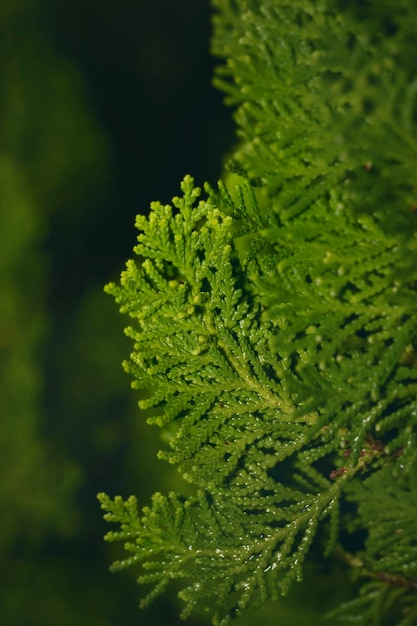This image captures a close-up view of the vibrant green, textured needle-like leaves of an evergreen plant, possibly a cedar or Leyland Cypress, set against a blurred black and green background. The plant's foliage forms a dense and flattened cluster, with some branches extending upwards, while others point downwards, creating a full and vibrant appearance that occupies about half of the frame. Clear, white droplets of moisture are visible on some of the leaves, adding a glistening effect to the detailed, somewhat sharp needle structure. In the background, blurred silhouettes of similar trees can be faintly discerned, emphasizing the focus on the detailed, foreground plant. The overall scene suggests a nighttime or low-light setting, illuminating the plant's bright green leaves against the dark backdrop.